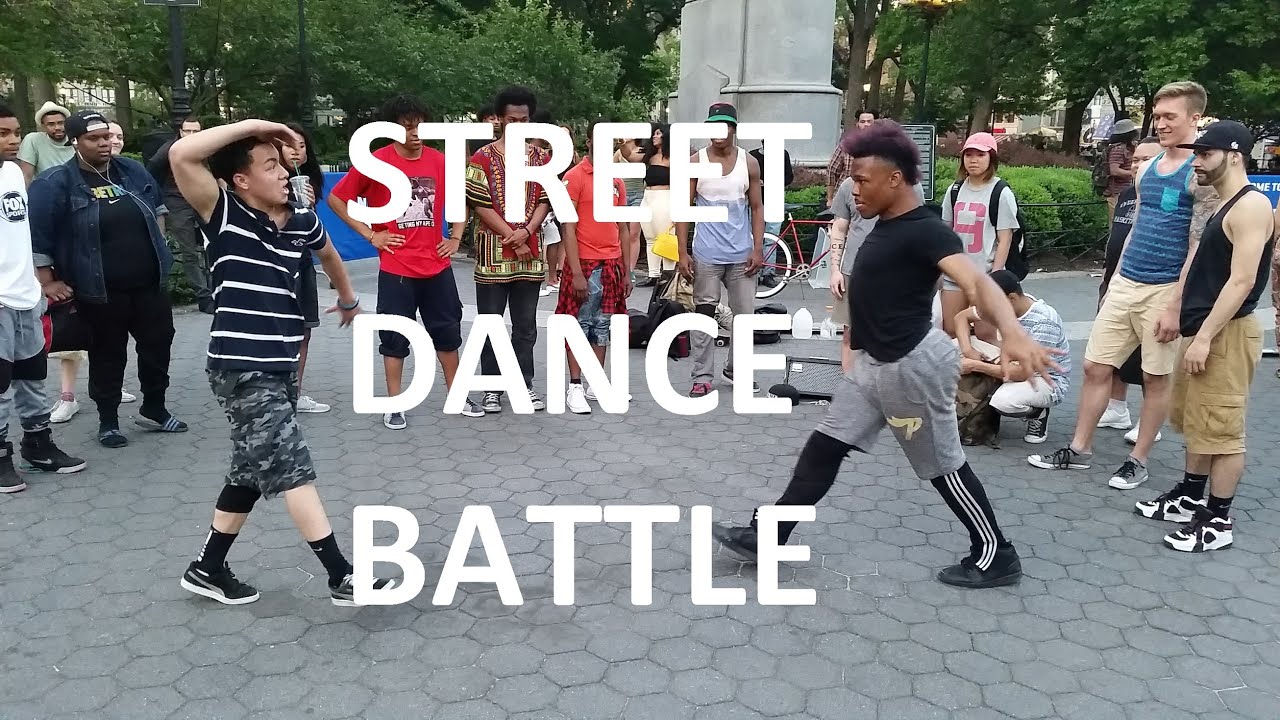In this captivating photograph, a Street Dance Battle unfolds in what appears to be a city center with hexagonally shaped paving blocks and a portion of a monument visible in the background, framed by trees. Bold white text centrally overlays the image, reading "Street Dance Battle" in three stacked lines: "Street" on top, "Dance" in the middle, and "Battle" at the bottom. 

The two central figures are young black men, possibly in their late teens to early twenties, deeply immersed in their dance moves. The person on the left, with a lighter skin tone, sports a blue and white striped polo shirt, camo shorts, black socks, black sneakers, and a knee pad on his left knee. He has his arms overhead, seemingly poised to start his routine, balancing on a single leg.

On the right, another dancer with distinctive purple, puffy hair, dons a black t-shirt, gray shorts over long black striped workout pants, and black sneakers. His arms are flailed back, and he too appears to be caught mid-dance, engrossed in the battle. Both dancers’ right legs are extended forward, contributing to the dynamic and energetic atmosphere.

Encircling the dancers is an enthusiastic crowd, their expressions ranging from amusement to keen interest, suggesting the impromptu event has captured their attention. The entire scene exudes a lively, spontaneous vibe typical of street dance battles, making it an engaging and electric moment frozen in time.